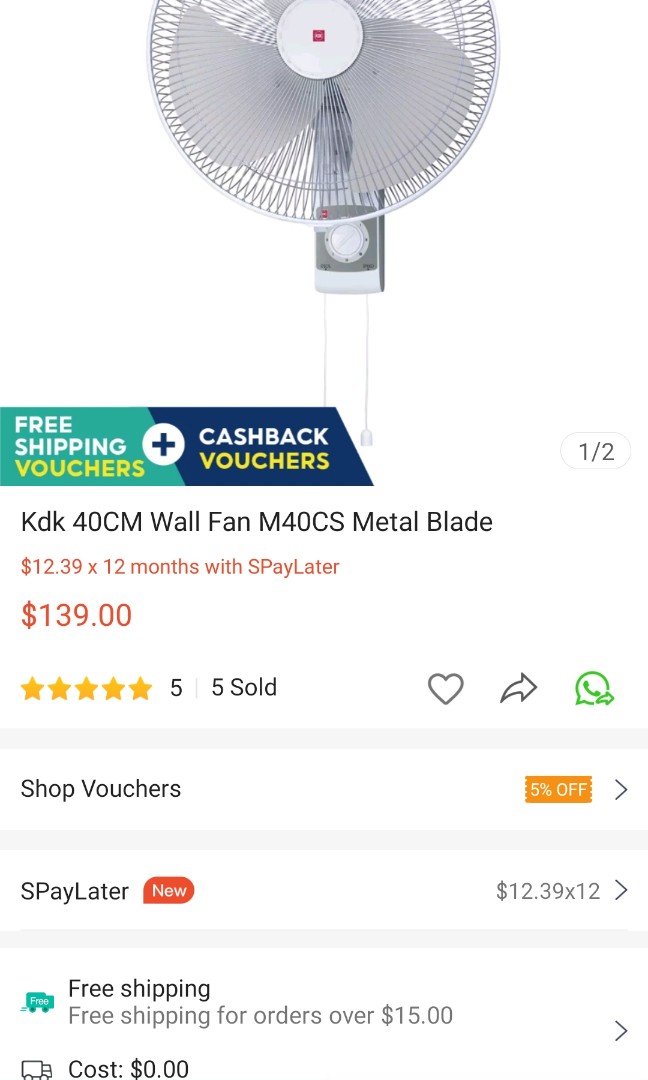This image showcases a listing from a website selling a white floor fan. At the top of the image, there is a clear picture of a pristine, sleek white fan. Below the image of the fan, there is a small informational box divided into two sections: the left side is green and the right side is blue. The green section mentions "Free Shipping Vouchers" with a plus sign, while the blue section states "Cashback Vouchers."

The product is identified as the KDK40CM Wall Fan with M40CS Metal Blade. The listing offers the option to purchase the fan via SP Pay Later at a rate of $12.39 per month for 12 months, totaling $139. The product has received a perfect 5-star rating, based on 5 sales.

Next to the fan’s name and pricing details, there are icons for saving the item to a wishlist (heart icon), sharing the product (arrow icon), and seeking customer service (telephone icon). Below these icons, there is a prompt to "Shop Vouchers," which includes a 5% discount indicated by an arrow. 

Further down, the image mentions SP Pay Later again, with a small box marked "New," reiterating the $12.39 monthly cost over 12 units. Additionally, it highlights the benefit of free shipping for orders over $15, confirming that the shipping cost will be zero.

The detailed layout ensures that potential buyers are well-informed about the product, pricing options, discount opportunities, and additional support features.